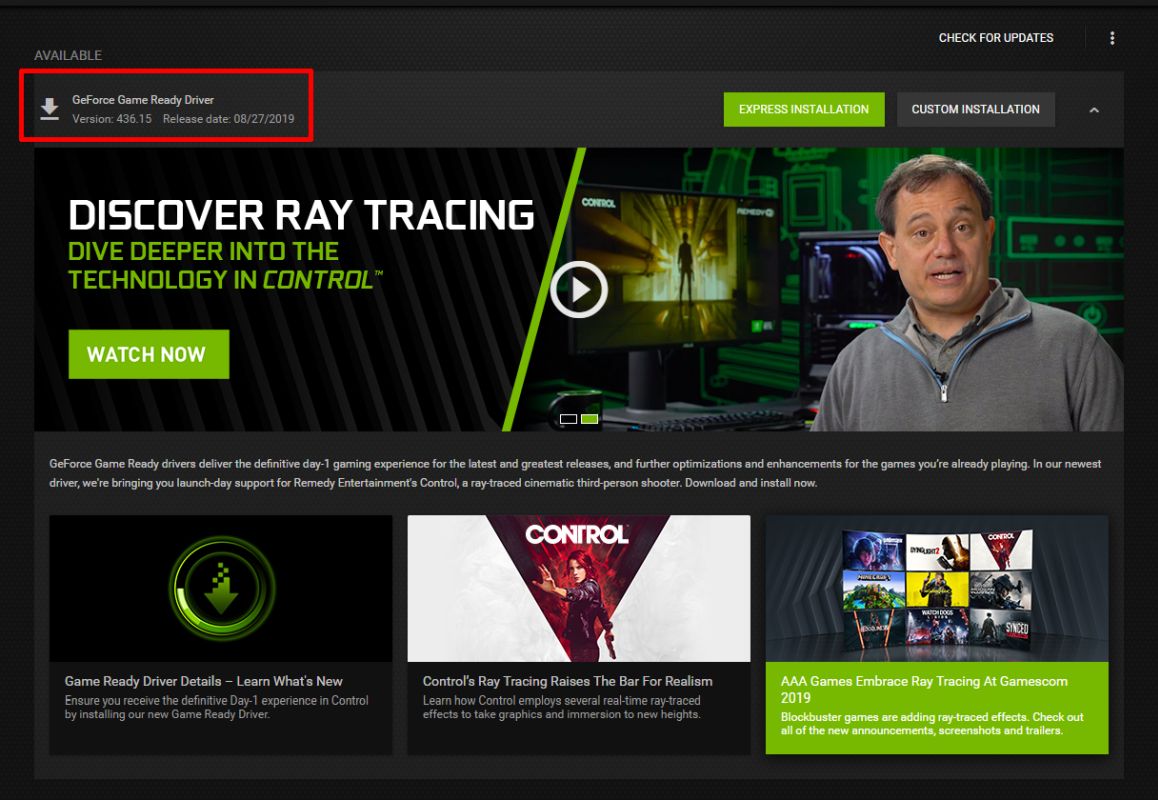The image depicts a website where users can download drivers, including game drivers, and explore new technology products. At the top, a black navigation panel features an option on the right labeled "Check for Updates." Below, a lighter gray panel has a section highlighted with a red box indicating the "GeForce Game Ready Driver," a key focus for downloading. Next to this section, there are two installation options: a green button for "Express Installation" and a grey button for "Custom Installation."

Further down, a large central panel showcases an image of a man standing beside a computer screen, with text on the left inviting users to "Discover Ray Tracing, Dive Deeper into the Technology and Control." This call-to-action is presented in green text, and a green "Watch Now" button in white text is located beneath the description, linking to a video. Below this large panel are three smaller rectangular panels: one detailing the game-ready driver, another discussing how ray tracing raises the bar for realism, and the third highlighting how AAA games embrace ray tracing.